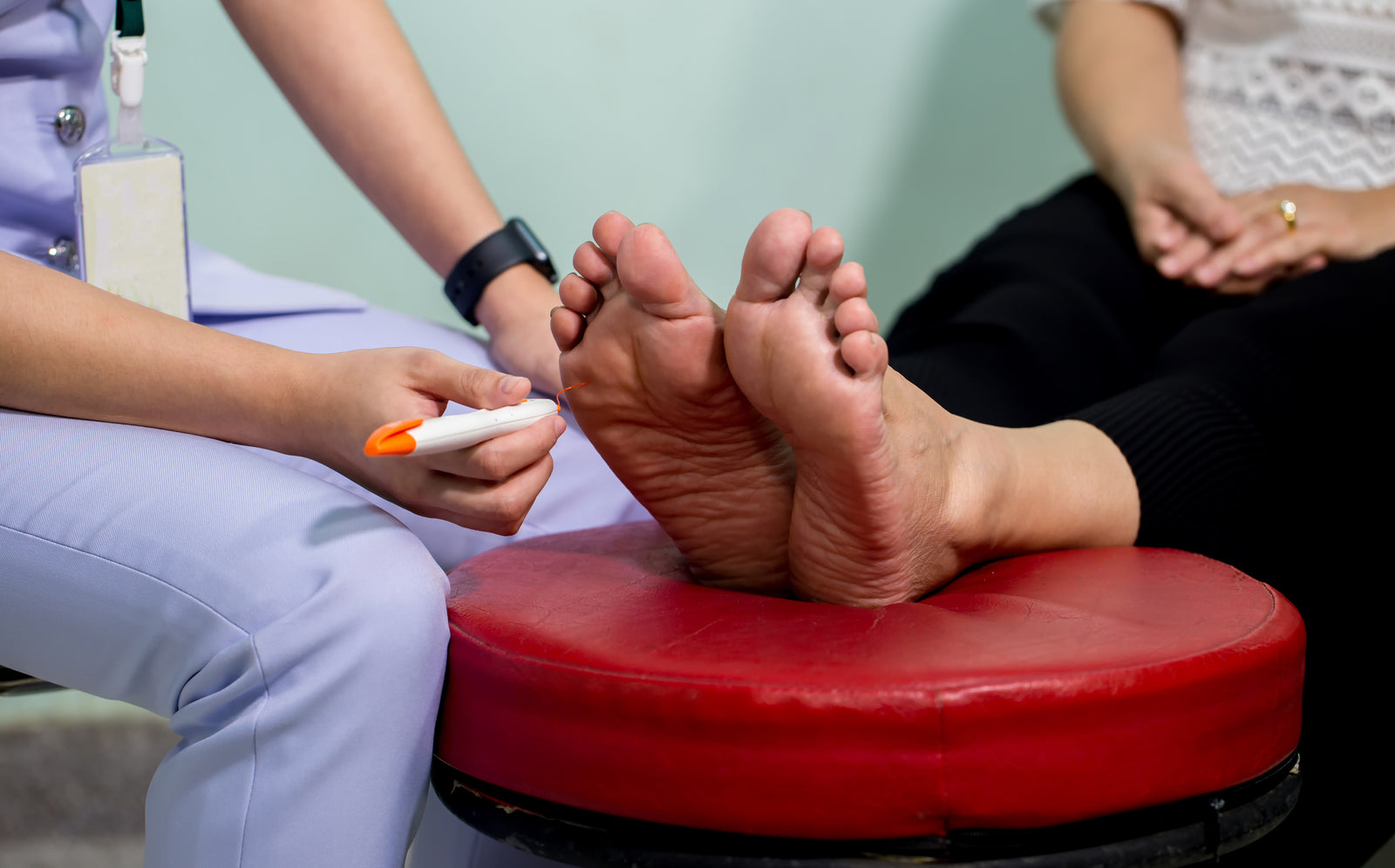The image captures a close-up scene of a medical examination, focusing on the lower bodies of two individuals. On the right, a woman is seated with both feet resting on a round, cushioned red stool, her heels turned upward and pressing into the cushion, creating noticeable impressions. She is dressed in a black skirt and a beige, short-sleeve top, with her hands clasped together, displaying a wedding band on one of her fingers. On the left side of the image, a medical professional is seated, wearing light blue scrubs and a lanyard with an ID that is not fully visible. The professional's left arm rests on their knee, adorned with a smartwatch, while their right hand holds a white tool with an orange cap and a thin probe extending from it, which is in contact with the sole of the woman's foot. The shot excludes both individuals' faces, focusing solely on the examination area.